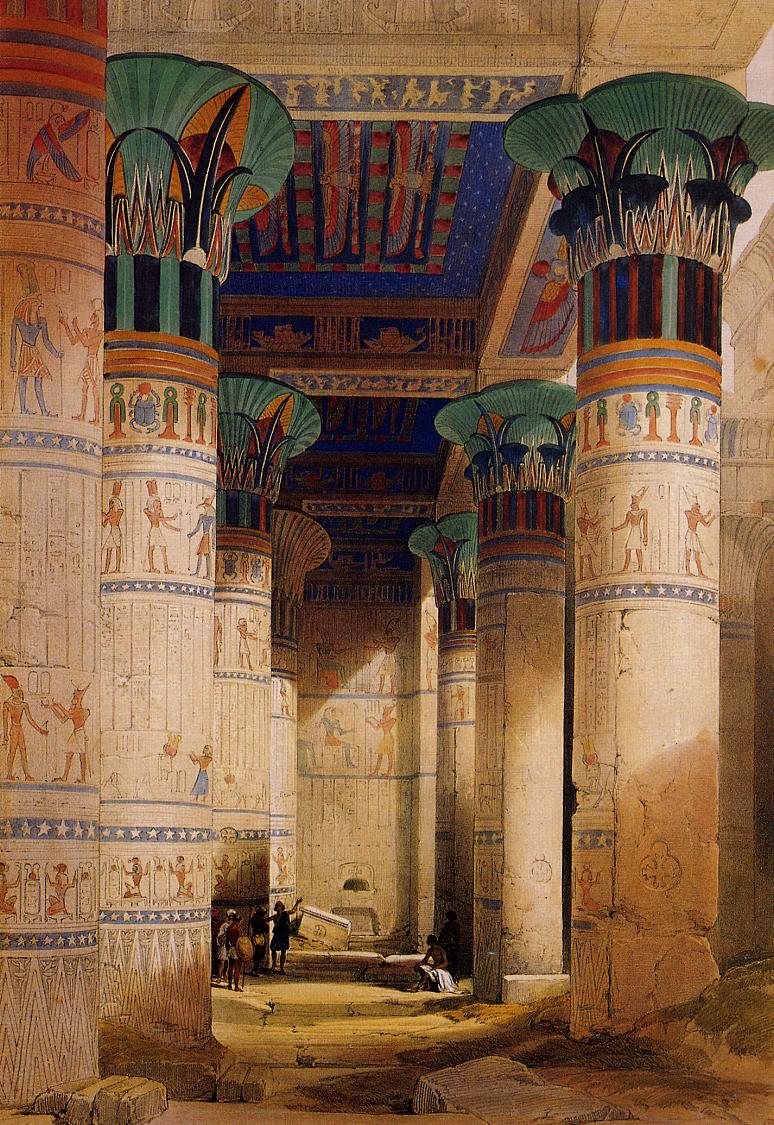This intricate painting depicts a grandiose Egyptian structure, likely a tomb or palace, featuring massive ornate columns that rise majestically to support a beautifully decorated vaulted ceiling. The pillars are adorned with elaborate designs, hieroglyphics, and images of Egyptian gods, showcasing an array of vibrant colors including blue, red, and light blue. The ceiling and walls are also richly painted, detailing various aspects of Egyptian history and art. The floor, possibly wooden with small steps, stands bare except for dirt, vegetation, and fallen stones scattered throughout, suggesting a place aged and partially ruined. Amidst this scene are several people: some standing, seemingly absorbed in conversation or study, while others sit near the walls, one with a cloth draped over his lap and another holding a shield. The setting is further enriched by an altar in the background and remnants of destroyed walls and pillars, adding a sense of historical decay to the majestic yet deteriorated environment.